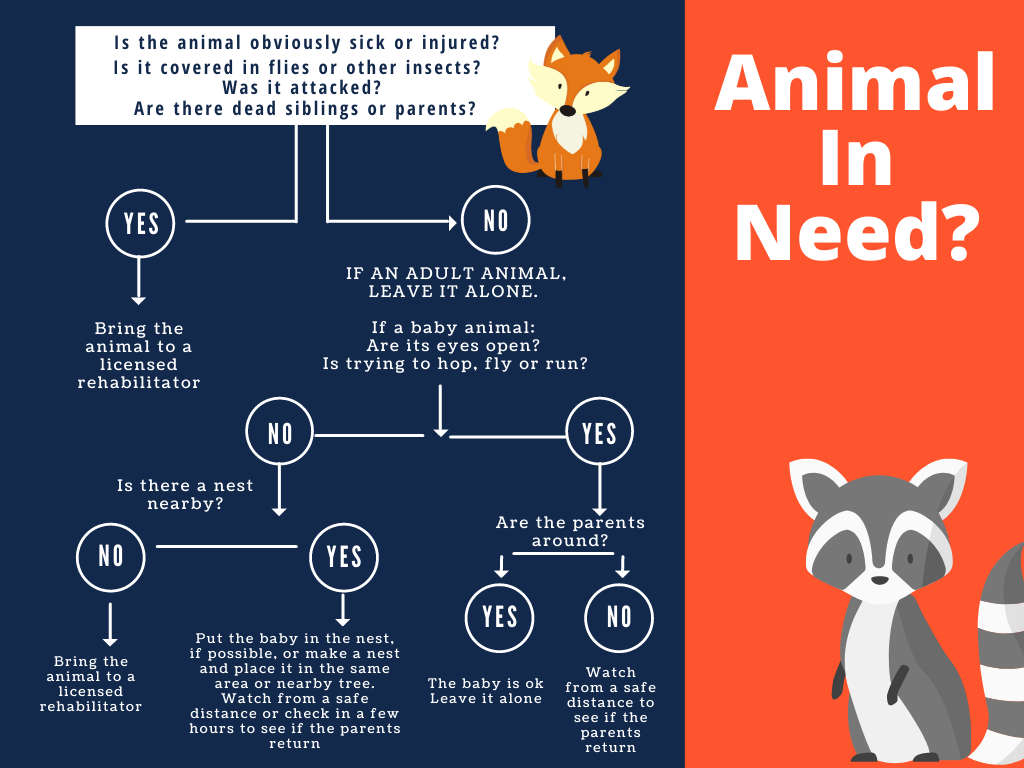This infographic provides a clear, step-by-step guide on what to do if you encounter a wild animal, focusing specifically on assessing whether the creature is sick, injured, or in need of assistance. The left portion, occupying about 60% of the visual space, features a dark blue background. At the top is a white rectangle with black text posing crucial questions: "Is the animal obviously sick or injured? Is it covered in flies or other insects? Was it attacked? Are there dead siblings or parents?" Next to these questions is an adorable illustration of an orange fox, adding a touch of whimsy. Below the questions, the flowchart begins with a "yes" or "no" option. If "yes," the instruction is clear: "Bring the animal to a licensed rehabilitator." For a "no" answer, the guidance diversifies: if the animal is an adult, you should leave it alone. If it's a baby and its eyes are open or it’s trying to hop, fly, or run, further assessment is required, including checking if there's a nearby nest and if the parents are around. The infographic suggests detailed steps, such as placing the baby back in its nest or creating a makeshift one, and advises on what to do if the parents are not observed to return. The right side of the image features an orange background with white text reading "Animal in Need," above a charming vector illustration of a gray and white raccoon, making the message both engaging and informative.